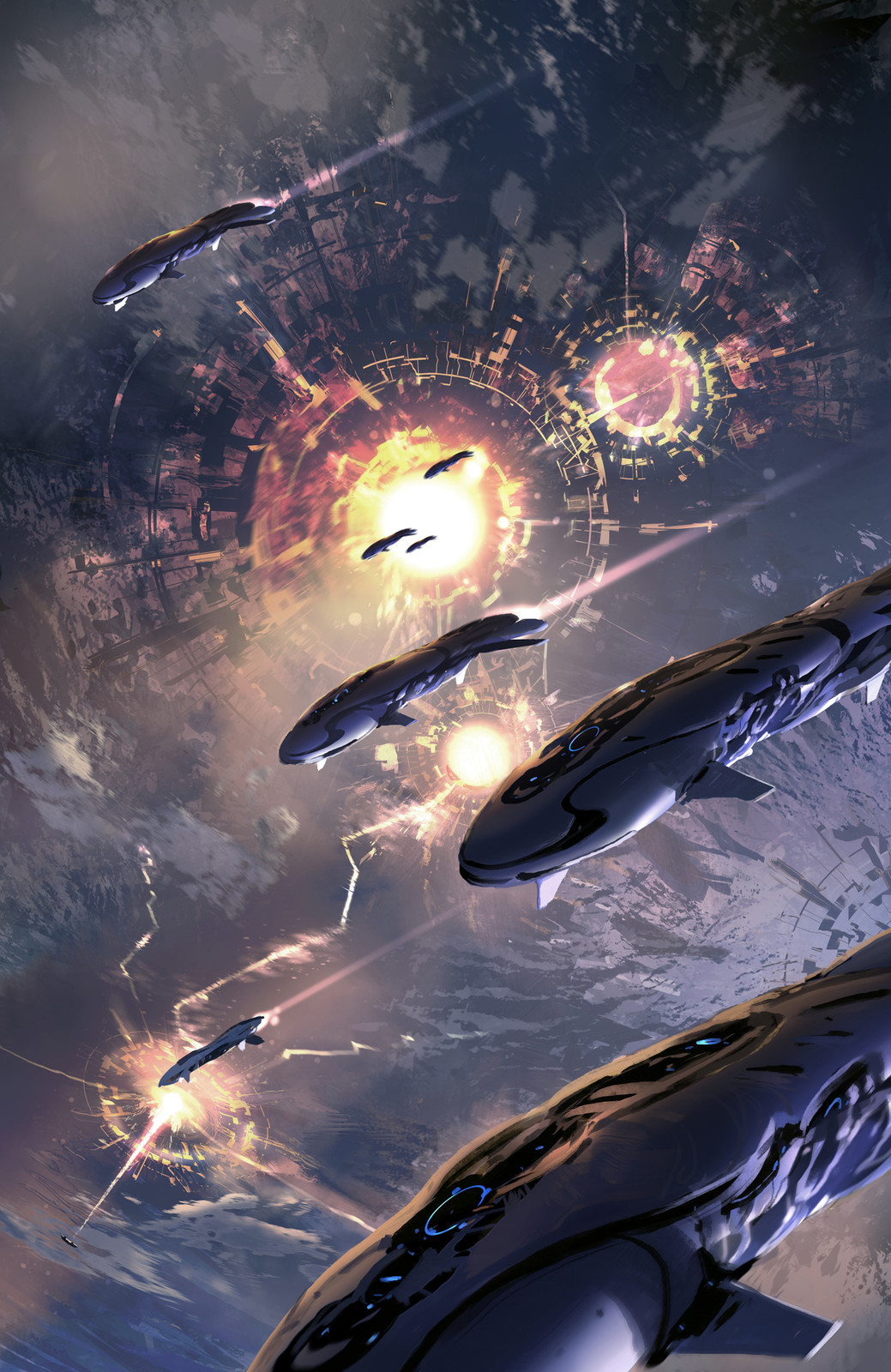This image appears to be a screenshot from a video game, likely depicting a cutscene given the cinematic camera angle and composition. The scene has a distinct sci-fi aesthetic featuring what look like large, whale-shaped spacecraft soaring through the sky. These ships resemble whales with their curvy front ends and small, fin-like structures on the sides.

The setting below shows a dramatic landscape, dominated by a large, fiery crater that suggests a significant impact or explosion has occurred. This central explosion is circular in shape, with flames and debris radiating from it. A smaller, secondary impact site is visible to the right, characterized by a red hue but lacking visible flames.

The overall atmosphere suggests a scene of conflict or battle, with the whale-like ships possibly engaged in an assault on the ground structures. The details and the dynamic perspective hint at a high-stakes moment in the game, filled with tension and destruction. The image's proportions suggest it might have been captured on a smaller screen, like that of a smartphone.